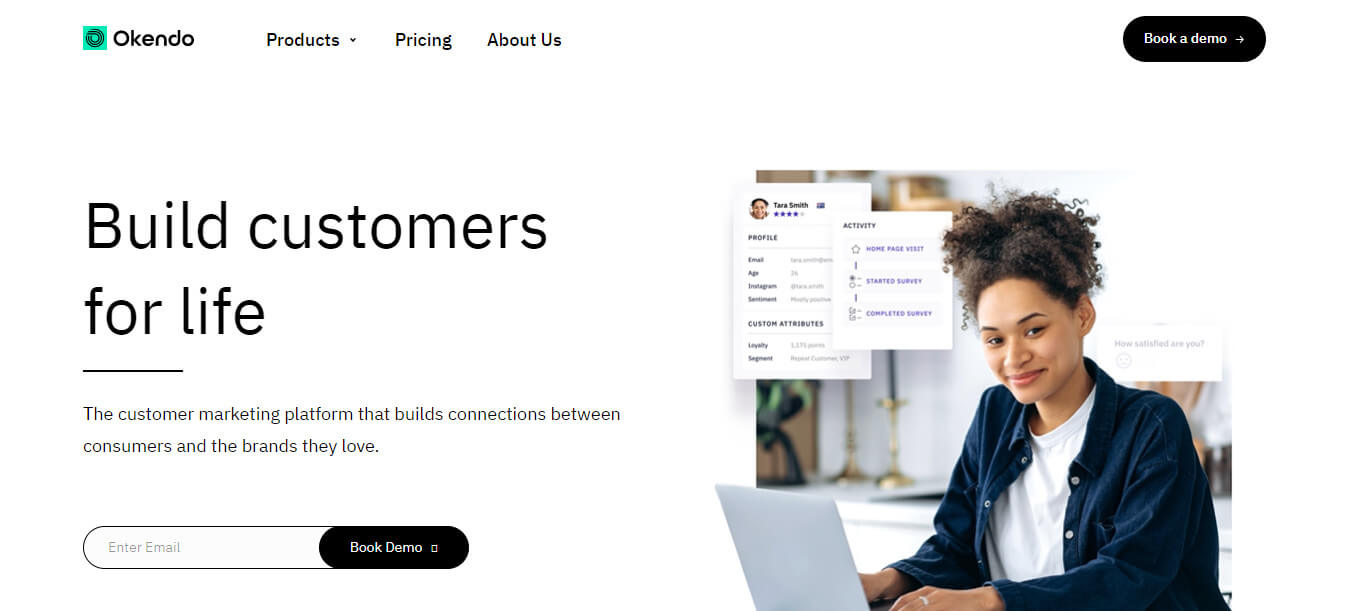This is a cropped screenshot of the Okendo home screen from their website. At the top left corner, the Okendo logo is prominently displayed. To the right of the logo, three categories are listed in small black letters: "Products," with a downward-pointing triangle indicating a dropdown menu for subcategories; "Pricing" in the center; and "About Us" to the right. On the far right side, there is a noticeable black button with white text that reads "Book a Demo," accompanied by an arrow pointing to the left.

At the bottom right of the screenshot, there is an enlarged thumbnail of a young woman using a laptop. Above her head, two white boxes display reviews and star ratings, as well as her performance metrics. On the left side of the image, the phrase "Build Customers for Life" is written in large black font. Below this, a smaller description is provided, followed by an email input box on the lower left. To the right of the input box, another "Book a Demo" call-to-action is visible.